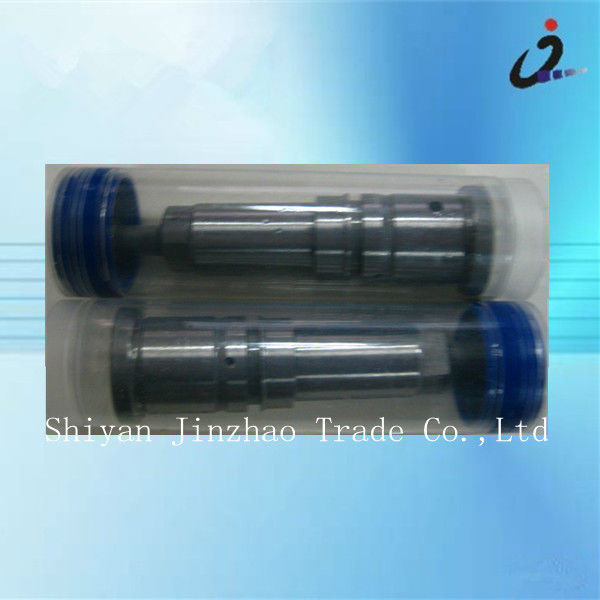The image features a turquoise background with shades of blue and multi-colored elements. In the upper right corner is a black logo resembling a squiggly doodle or a backward 'C' with a red dot on top and some navy blue triangular elements below. The main focus of the image is a pair of vertically stacked, cylindrical canisters with plastic exteriors and metallic or gray centers, each enclosed in a clear casing. The canister on top has a blue circular cap on the left and a white cap on the right, while the one on the bottom features a white cap on the left and a blue cap on the right. Underneath the canisters, white text reads "Xi'an Jinzhao Trade Co. Ltd."